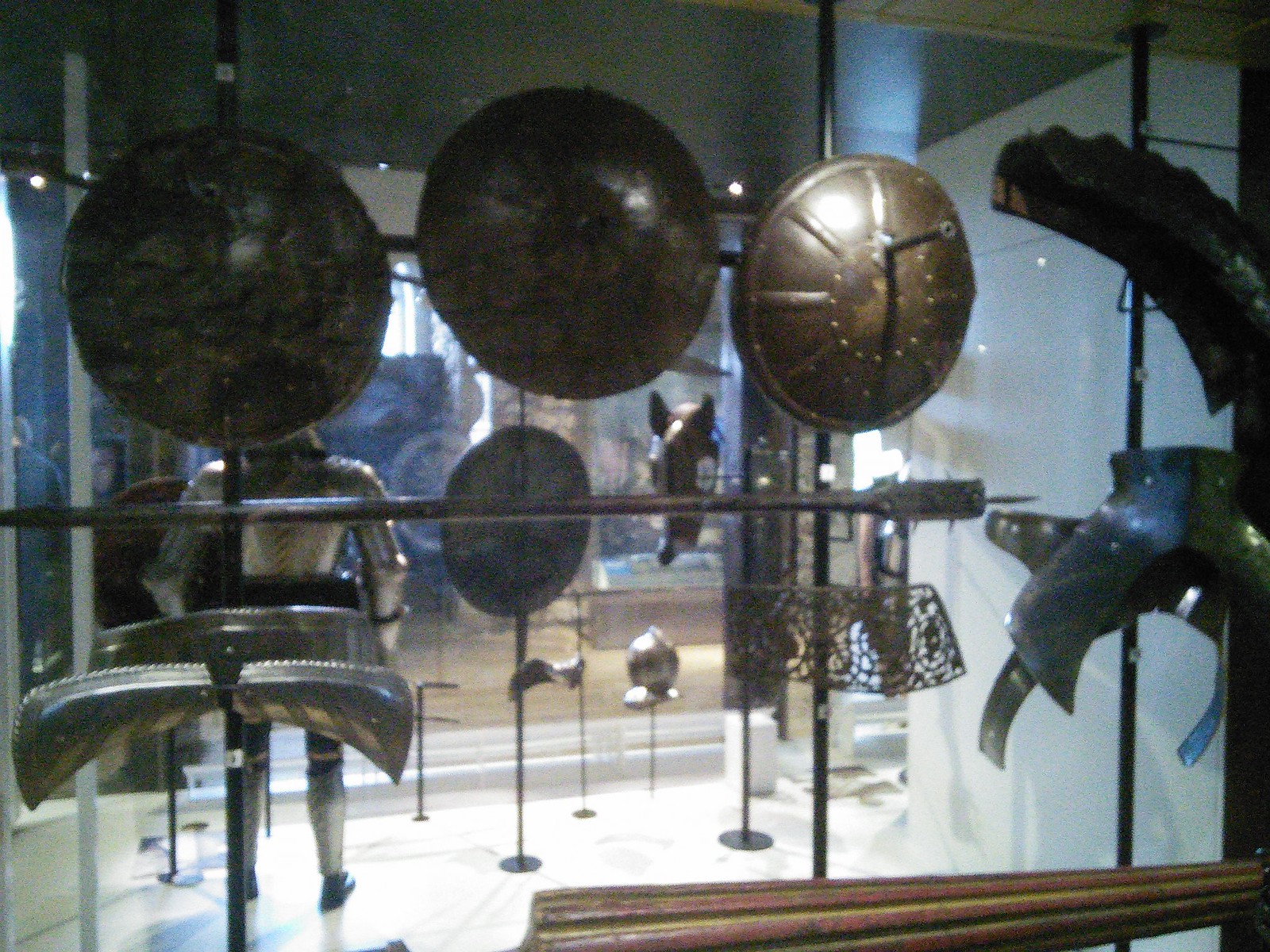This image depicts a detailed exhibit of medieval weaponry and armor. In the foreground, there are three bronze shields displayed from left to right, with the rightmost shield pierced by a pole. Below it, a dark gray shaft extends forward, tipped with a blade, and features a mustache-shaped ridge with hard curves at the bottom. A white floor contrasts with the white wall on the right side of the image. In the background, a reflective surface reveals a suit of silver metal armor with articulated arms, legs, and chest. Black bars run vertically, supporting the ceiling. There are various other objects, including what appears to be a horse's head, a man in armor, a helmet, swords, and a large wooden rectangular piece, adding to the complexity and richness of the exhibit.